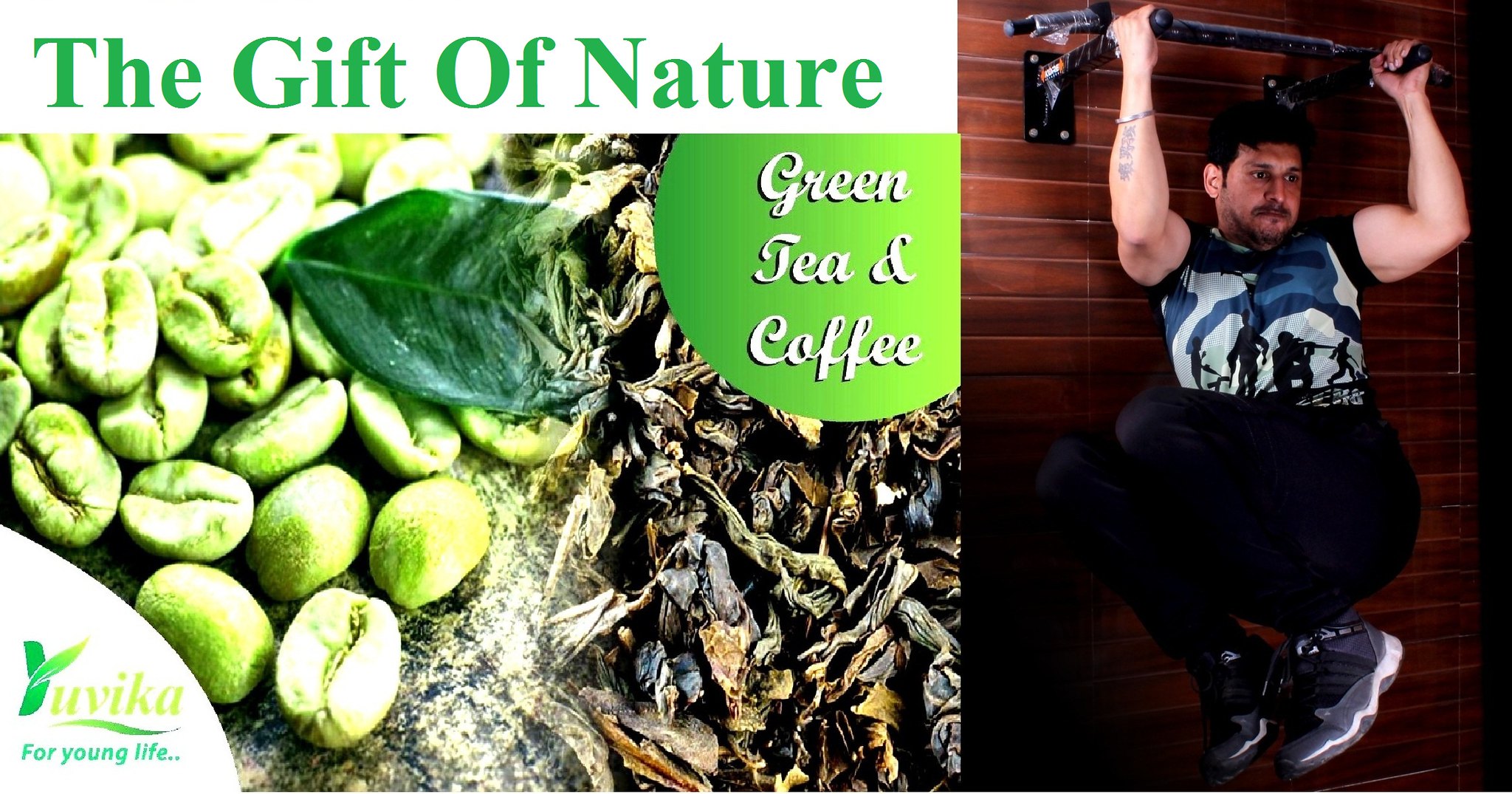The image captures a compelling health advertisement, likely for a natural food store or gym, featuring a harmonious blend of elements that celebrate both fitness and natural products. Approximately three-quarters of the image is bathed in a greenish tint, emphasizing "The Gift of Nature: Green Tea and Coffee." Displayed prominently are greenish-white coffee beans accompanied by a leaf and some brownish tea leaves. On the lower left-hand side, the site name "UVica," partially rendered in green with the rest in yellow, is displayed, with the tagline "For Young Life" beneath it. To the right, a muscular young man is intensely engaged in a pull-up workout at a gym. He sports a camouflage-patterned dark tank top, black pants, and sneakers, underscoring a robust, active lifestyle. The image seamlessly marries elements of natural wellness and physical fitness, appealing to individuals dedicated to health and vitality.